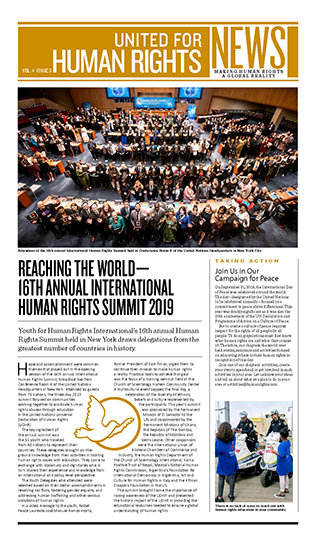The image is a detailed newsletter or newspaper featuring a prominent gold banner across the top with the white text "United for Human Rights." Positioned below it is a white box with the word "NEWS" in yellow, alongside smaller print. Dominating the top section of the publication is an overhead image of a large, formal conference, likely the United Nations, showing numerous men and women seated at circular desks.

On the left side of the page, two columns of text are introduced with the headline "Reaching the World: 16th Annual International Human Rights Summit 2019." The article goes on to describe the Youth for Human Rights International's summit held in New York, which drew the most country delegations in its history.

To the right, another smaller headline reads "Join us in our Campaign for Peace," followed by a few paragraphs elaborating on the campaign. Near the bottom of the page, a picture shows two police officers on motorbikes alongside an adult and a child, both wearing blue outfits that extend to their knees, suggesting some form of peaceful protest or event.

This combination of visuals and detailed articles encapsulates a comprehensive view of international efforts and events geared towards promoting human rights and peace.